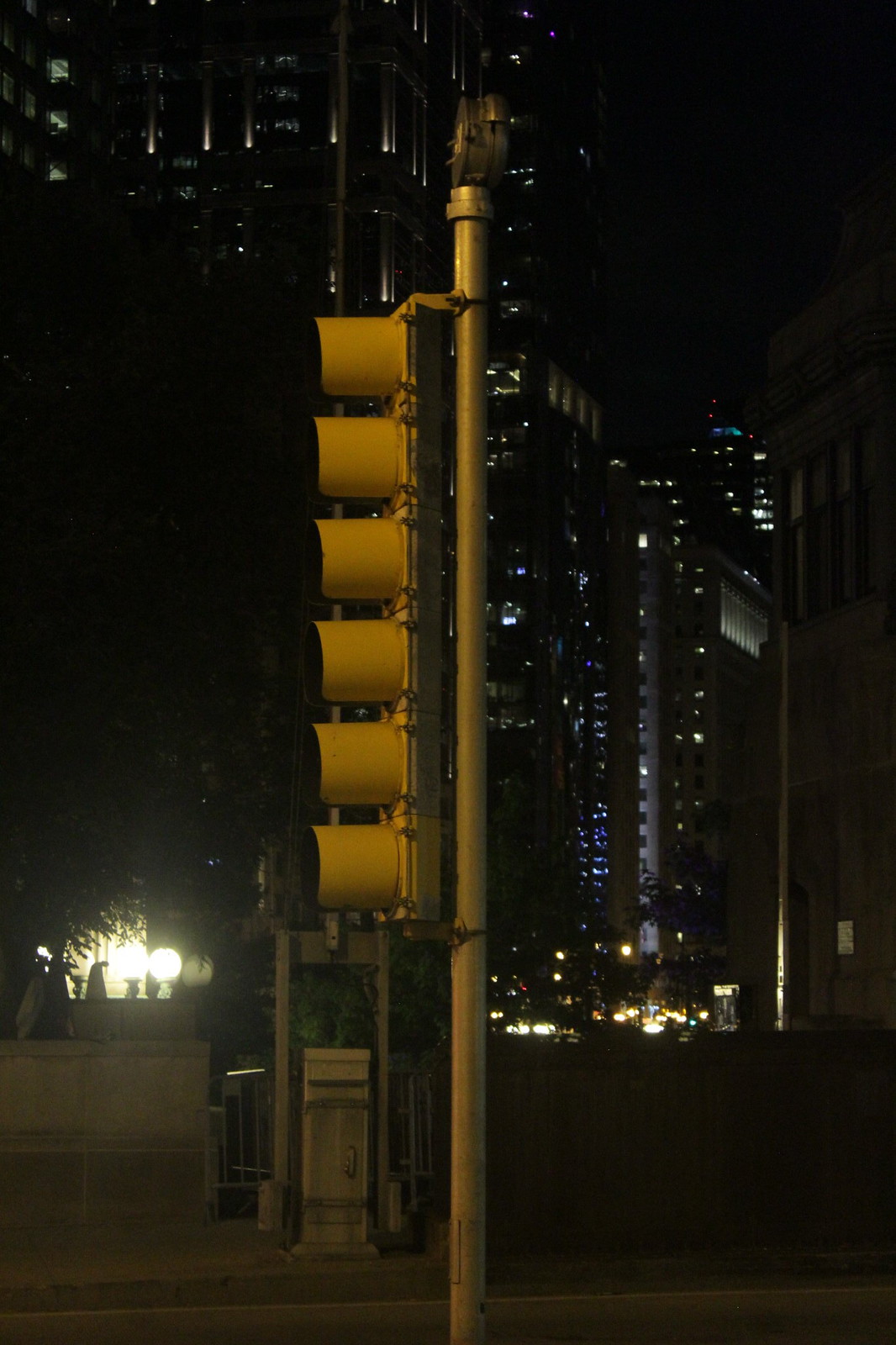The image is a color photograph capturing a nighttime urban scene. Dominating the center is a silver pole extending up to 80% of the image, topped with a unique traffic light featuring six signal circles, all oriented roughly at the 8:30 to 9:00 direction. Perched on top of the pole is a black bird, facing the viewer but angled slightly towards 5:30. The background reveals a cityscape with commercial buildings and skyscrapers, some tens of stories high, sparsely lit by office lights and storefronts. The scene, possibly taken from one side of a road looking across, hints at car lights and streetlights, all against a pitch-black sky, providing a minimal yet striking illumination to the image.